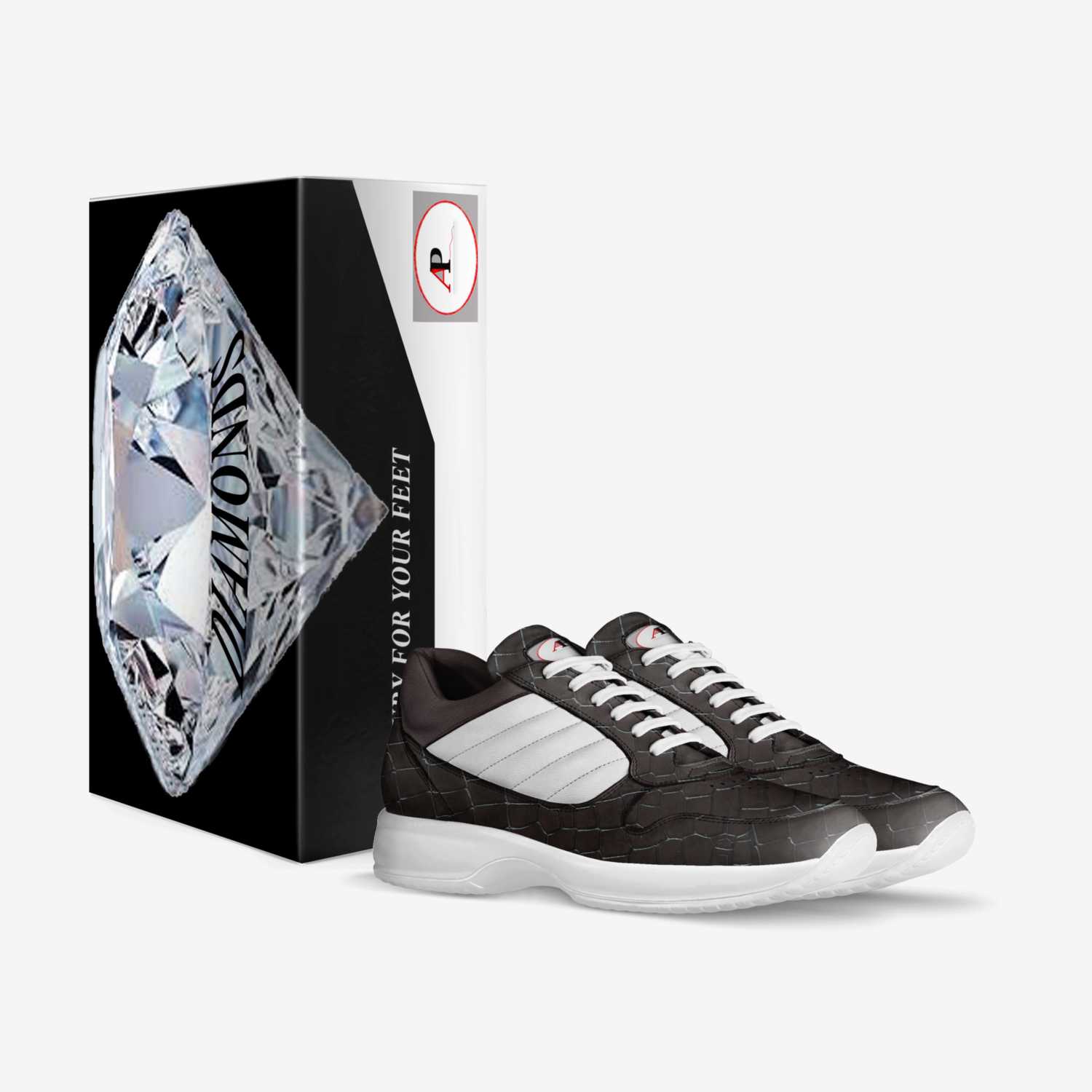The image displays a close-up of a pair of grey sneakers with distinctive white soles and white laces. They feature white stitching on the sides and white lines accentuating the grey portions. Notably, a dark brown leather band arches over the heel of each shoe, and the tongue bears a white oval logo outlined in red, with the letters "AP" inside – the A in red and the P in black. The sneakers also include a subtle red design detail. Behind the sneakers stands a vertically positioned box, predominantly black with a white base, adorned with an image of a large diamond. The diamond illustration is topped with the word "DIAMONDS" in bold, capitalized black letters, while the box features the phrase "For Your Feet" in white capital letters. The bottom right corner of the box displays a grey rectangle with the AP logo, mirroring the branding on the sneakers. The image clarity is high, with a bright, naturally lit white background, enhancing the sharpness and detail of the product features.